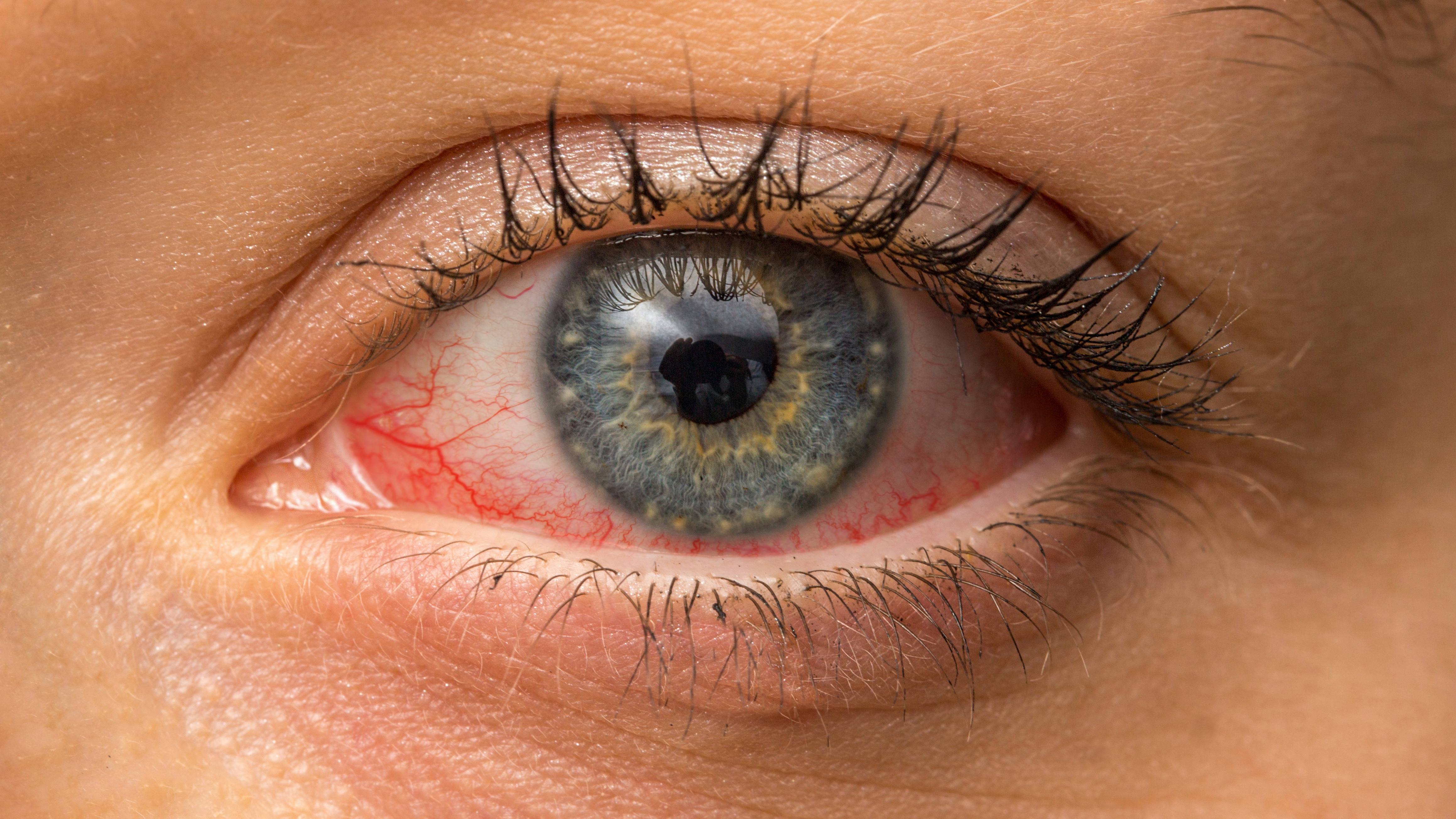This is an extreme close-up photograph of a light-skinned, presumably Caucasian individual's left eye, showcasing intricate details with remarkable clarity. The skin surrounding the eye has a peachy, light tan tone with visible pores, and fine lines suggestive of aging. The upper right corner reveals the tail end of a carefully groomed eyebrow. The long, black mascara-enhanced eyelashes are notably curled, ensuring they do not obscure the view of the iris and cornea. Both the top and bottom lashes are distinctly visible. The sclera, or white part of the eye, is prominently bloodshot with numerous red veins. The iris exhibits a striking gray color interspersed with cloudy orange and yellow striations, resembling muscle fibers or clouds, radiating outwards. The pupil, neither overly dilated nor constricted, contains a reflection of the person holding a camera to capture this detailed image.